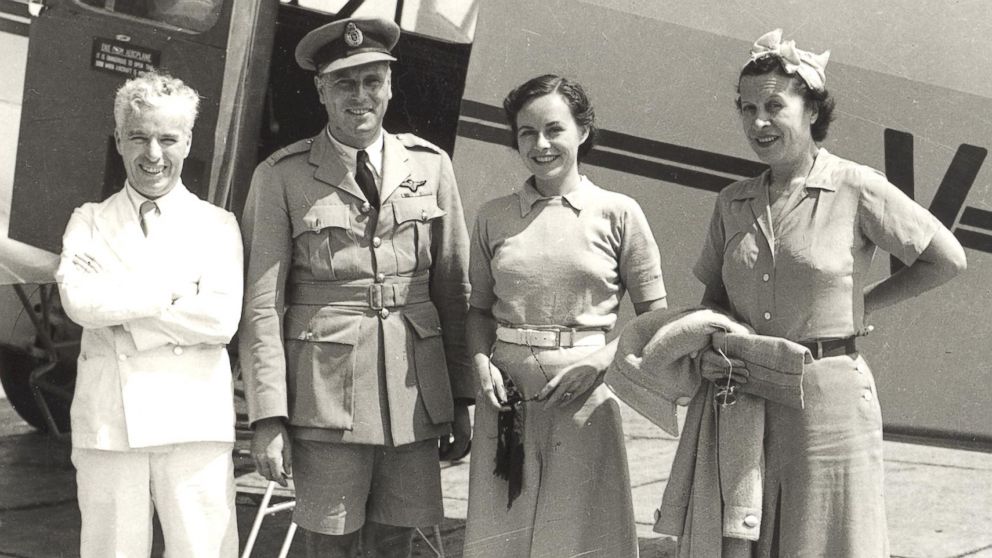This is a detailed, black-and-white photograph in landscape layout, showing four Caucasian individuals posing in front of a white airplane with its back door open. The photograph, visible from their knees upwards, depicts the following from left to right:

The first individual, an older gentleman, is dressed in a white suit with a light-colored, buttoned-up coat and a tie. He is clean-shaven and smiling directly at the camera.

Next to him stands a slightly younger and taller man in a military uniform. He is wearing a buttoned-up tunic coat with metal buttons, light-colored shorts ending above his knees, and a pilot's cap.

To the right of the men, there is a woman in a short-sleeve dress with a collar and a belt, smiling and holding a pair of sunglasses in her hands.

The fourth individual, another woman, is wearing a skirt and a buttoned-up top with a dark belt. She is holding sunglasses, a purse, and a jacket, with one hand positioned behind her back and a headband adorning her hair.

All four individuals, appearing to be in their 50s and 60s, are standing and posing confidently against the industrial backdrop of the airplane. The image conveys a historical vibe, likely capturing a moment from the mid-20th century.